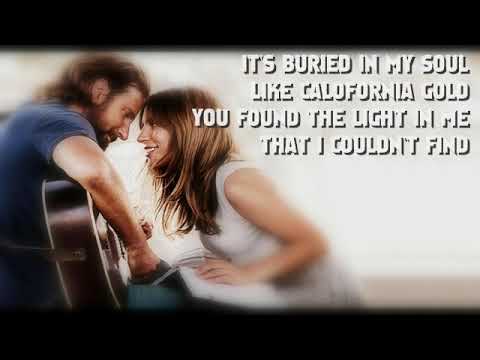The image displays a touching scene from the movie *A Star is Born* featuring Bradley Cooper and Lady Gaga. On the left side of the image, Bradley Cooper, with brown hair, a mustache, and a beard, is depicted playing a guitar while wearing a blue short-sleeved t-shirt. He faces Lady Gaga, who stands at the center of the image with her long brown hair and white sleeveless dress. Their foreheads are gently touching as they slightly smile at each other, creating an intimate moment between the two. The background features a dark border, and in the top right corner, white capital letters spell out the lyrics, "It's buried in my soul like California gold. You found a light in me that I couldn't find." The overall aesthetic, with its mix of black, white, brown, blue, and green hues, suggests an inspirational and romantic mood that is likely designed for sharing on social media.